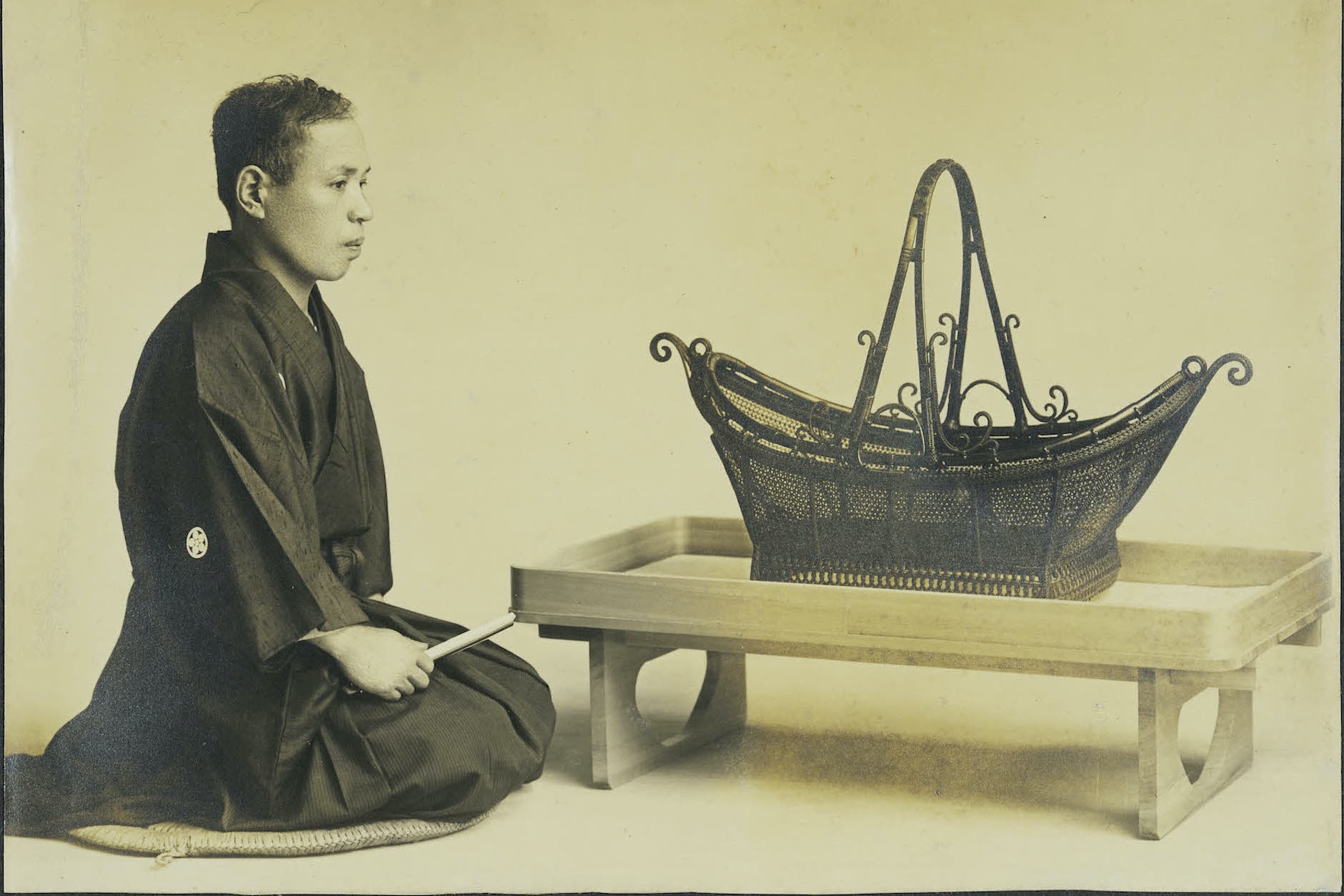In this grainy, old black-and-white photograph, a Japanese man is kneeling on a round woven tatami mat. He is dressed in a dark kimono, which features a small floral symbol on it, and his short black hair is neatly kept. From a right-side view, the solemn figure grasps an off-white rod or stick in his right hand, possibly a fan. The background is a plain beige color, emphasizing the subject. In front of him, a low, light-colored wooden table, resembling a coffee table only a few inches off the ground, holds a prominent intricate basket. This basket, dark and ship-shaped with narrow, curved ends and a big handle, contrasts sharply against the light wood of the table. The man gazes pensively at this basket, immersed in thought.